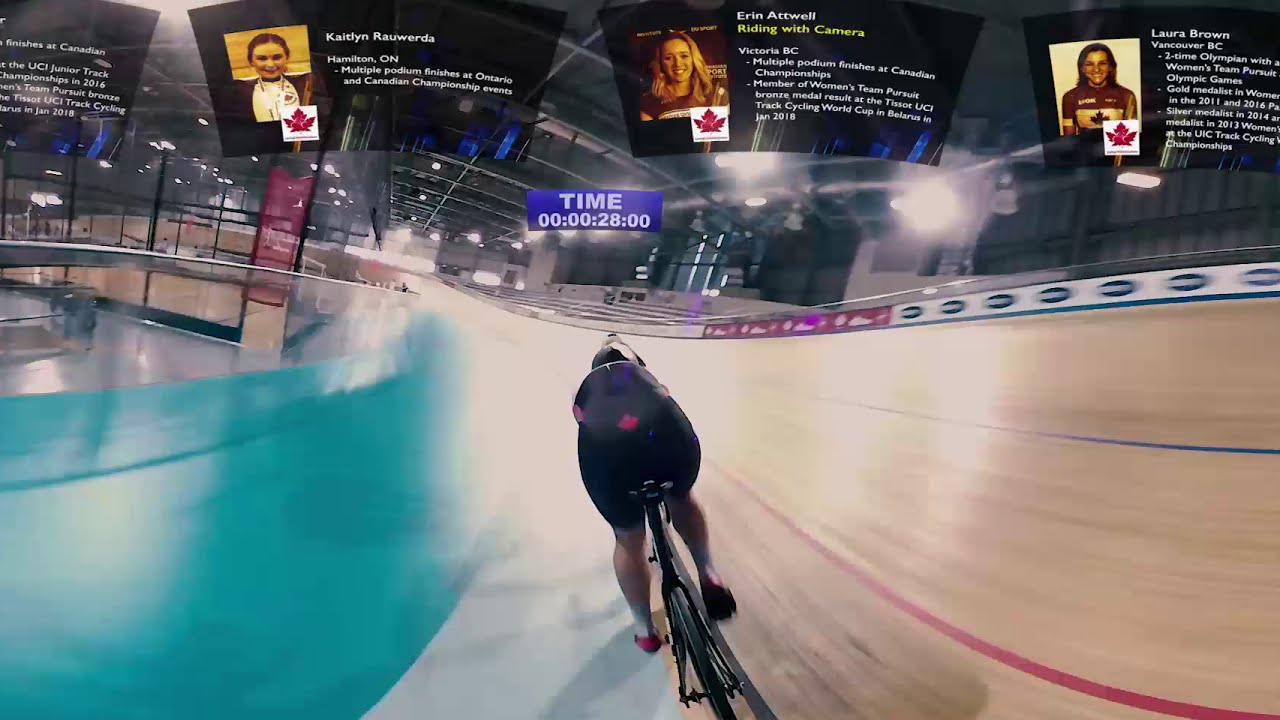A blurred photograph captures a dynamic scene inside an indoor bike racing arena. A cyclist, possibly female, clad in a black and red biking outfit, speeds along an inclined wooden track with lanes marked by red and blue stripes. To her left, the area is painted blue, while the stripes to her right blend into a pinkish-purple hue. Overhead, various signages and photographs of competitors are displayed, each accompanied by a Canadian maple flag. Notable names include 'Aaron Atwell, Victoria BC,' 'Caitlin Rwanda, Hamilton, Ontario,' and 'Lauren Brown.' A blue square sign reads 'TIME' with '28:00' on a clock. The intricate setup and vivid details reflect a professional indoor cycling event.